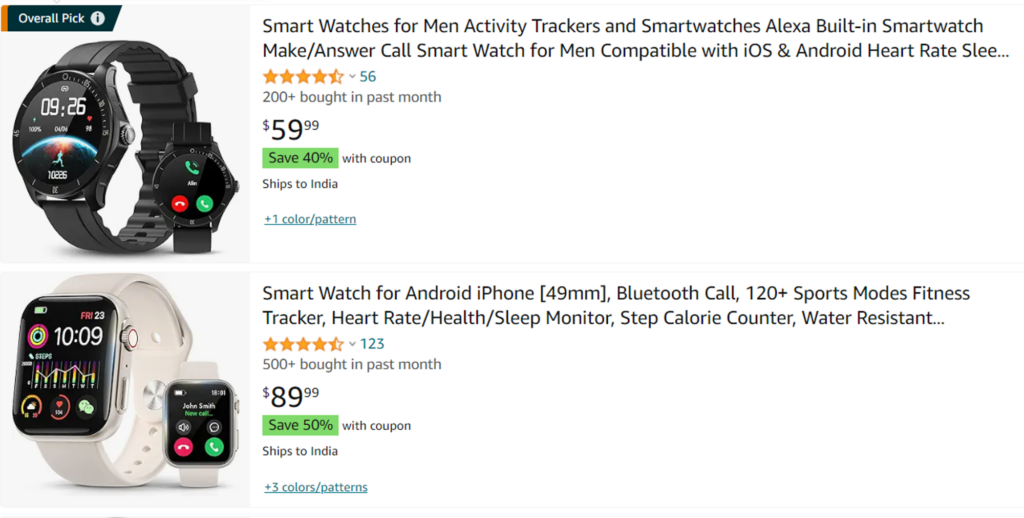Screenshot of an Amazon webpage displaying two smartwatches with their descriptions and prices.

The image has a white background with no border. At the top left corner, there is a blue banner that reads "Overall Pick." 

Below the banner, there are two watch listings:

1. At the top left, there is a black digital smartwatch. The description to the right reads:
   - "Smart Watches for Men, Activity Trackers and Smart Watches, Alexa Built-in, Smart Watch for Men Compatible with iOS and Android, Heart Rate, Sleep Monitor."
   - Rating: 4.5 stars
   - Price: $59.99
   - Additional info: "Ships to India" and "Save 40% off with coupon."

2. Below the first watch, there is another watch, this time gray with a rectangular screen displaying various digital icons. The accompanying description states:
   - "Smart Watch for Android and iPhone, 49mm, Bluetooth Call, 120+ Sports Modes, Fitness Tracker, Heart Rate, Health, Sleep Monitor, Step and Calorie Counter, Water-Resistant."
   - Rating: 4.5 stars
   - Price: $89.99
   - Additional info: "Save 50% with coupon" and "Ships from India."

Overall, the image displays online advertisements for two smartwatches, providing detailed information on features, pricing, and purchasing options.